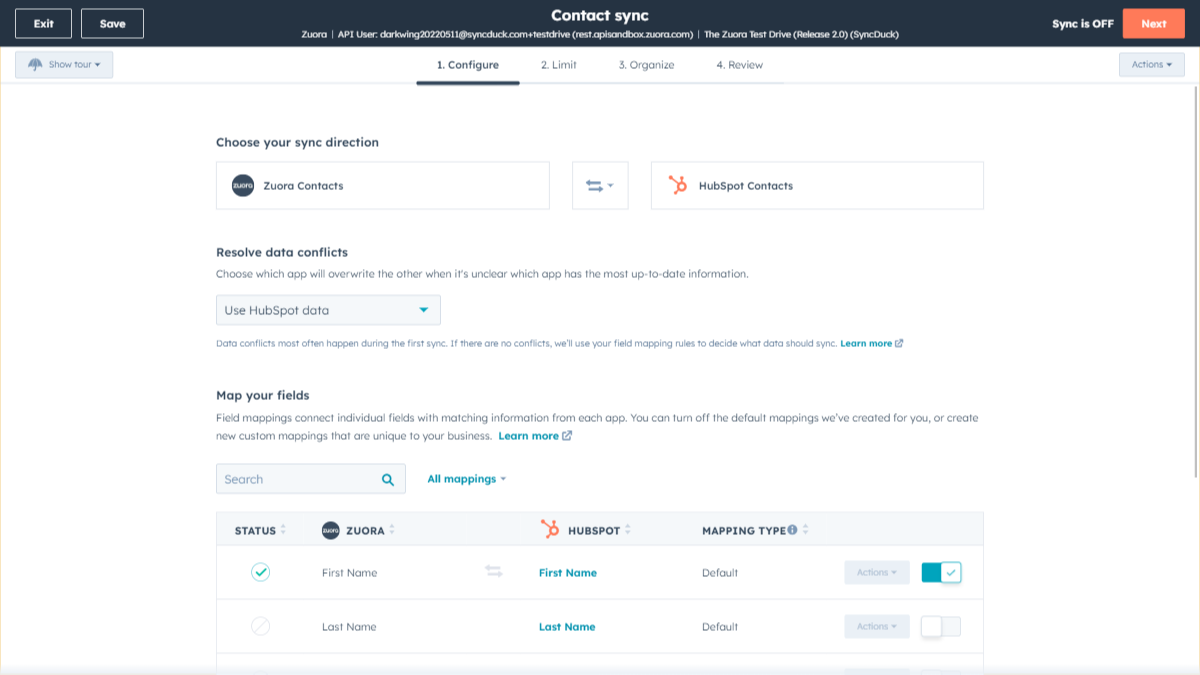The image depicts a web page interface for "Connect Sync." At the top, there is a black bar with "Connect Sync" prominently displayed. On the left side of this bar, there's an option labeled "Exit and Save," while the right side indicates that "Sync is Off." Below this header, a noticeable orange button labeled "Next" stands out.

The main interface is divided into several sections and categories. There's a title "Contact Sync," though the accompanying text is too small to decipher. The prominent categories listed below are "Configure," "Limit," "Organize," and "Review." The page allows users to select their sync direction between "ZUORA Contacts" and "HubSpot Contacts," with two blue arrows pointing left and right to indicate the sync direction options.

Beneath the sync direction, there's a section for "Resolve Data Conflicts," defaulting to "Use HubSpot Data," with a dropdown arrow to potentially change this setting. Another section labeled "Map Your Fields" follows, offering additional information and a search function. The mappings are categorized under "All Mappings," which include status indicators.

A checkbox system displays field mappings: one specific checkbox is marked, listed under "ZUORA," which appears to align with the first field named "First Home, First Name, Default." Directly opposite, under "HubSpot," the fields "First Name" and "Last Name" are shown in blue. The marked checkbox corresponds to the first bar across these categories.